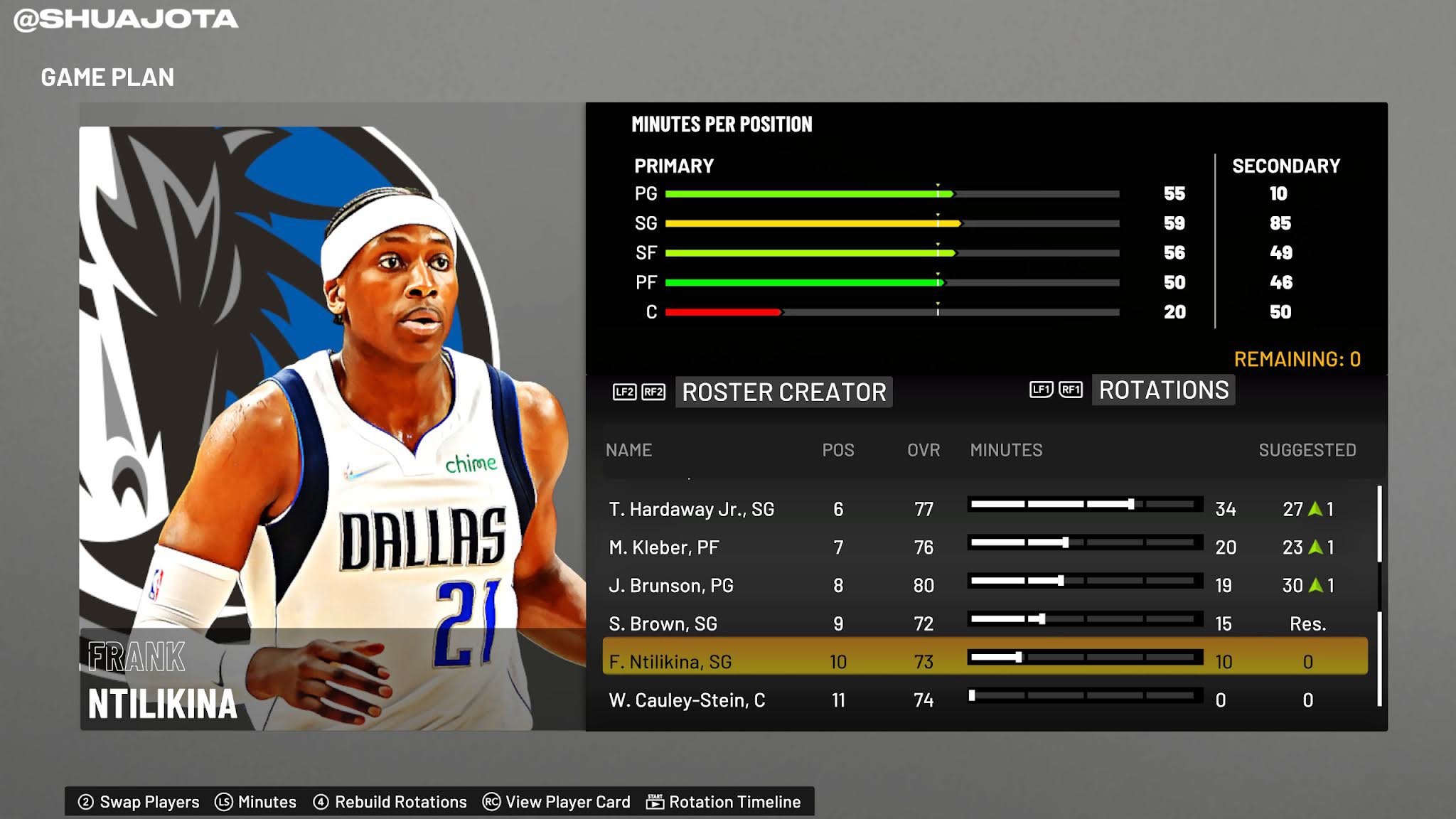This image is a detailed screenshot from a basketball video game, possibly within a fantasy setting. In the upper left corner, it features the user handle "@ShuaJota." The header of the screen reads "Game Plan."

The central focus of the image is a player from the Dallas Mavericks, identified as Frank Ntilikina. He is pictured wearing the team's jersey number 21, along with a white headband. The Dallas Mavericks logo is visible behind him. Frank Ntilikina, who might be of African descent, appears prominently in the image.

To the right of the player's image, there are detailed statistical charts and graphs. These graphs detail "Minutes per Position," listing primary and secondary roles such as point guard, shooting guard, and small forward. Notably, Frank Ntilikina scores a 20 for the center position, indicating a lower proficiency, while he scores a 56 for the point guard position, suggesting stronger performance in this role. 

Additional charts provide insights into the team's rotations and overall strength, mentioning players like Hardaway, Kleber, Brunson, and Brown. Each player's relative strength is depicted via bar graphs, alongside the minutes they play. This setup likely represents a meticulously managed team assembly in the game, possibly reflecting a blend of fantasy sports management and video gaming elements.